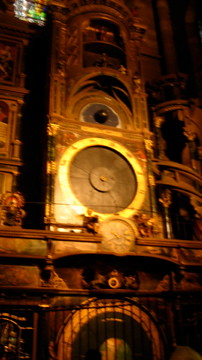This image features a distinctive wall clock embedded in a stone facade on the side of a building. At the bottom of the image, there is a black wrought-iron gate. The image appears to be a cropped section of a larger photograph. The wall around the clock is brown, with a golden border encircling the clock face, which itself is black with gold hands. Flanking the clock on both the left and right are decorative columns. Above the clock is a platform, and directly above that is an eye motif with white edges and a dark blue or gray iris with a black pupil at the center. Beneath the clock, there are small figures, resembling little people, adding intricate detail to the scene.